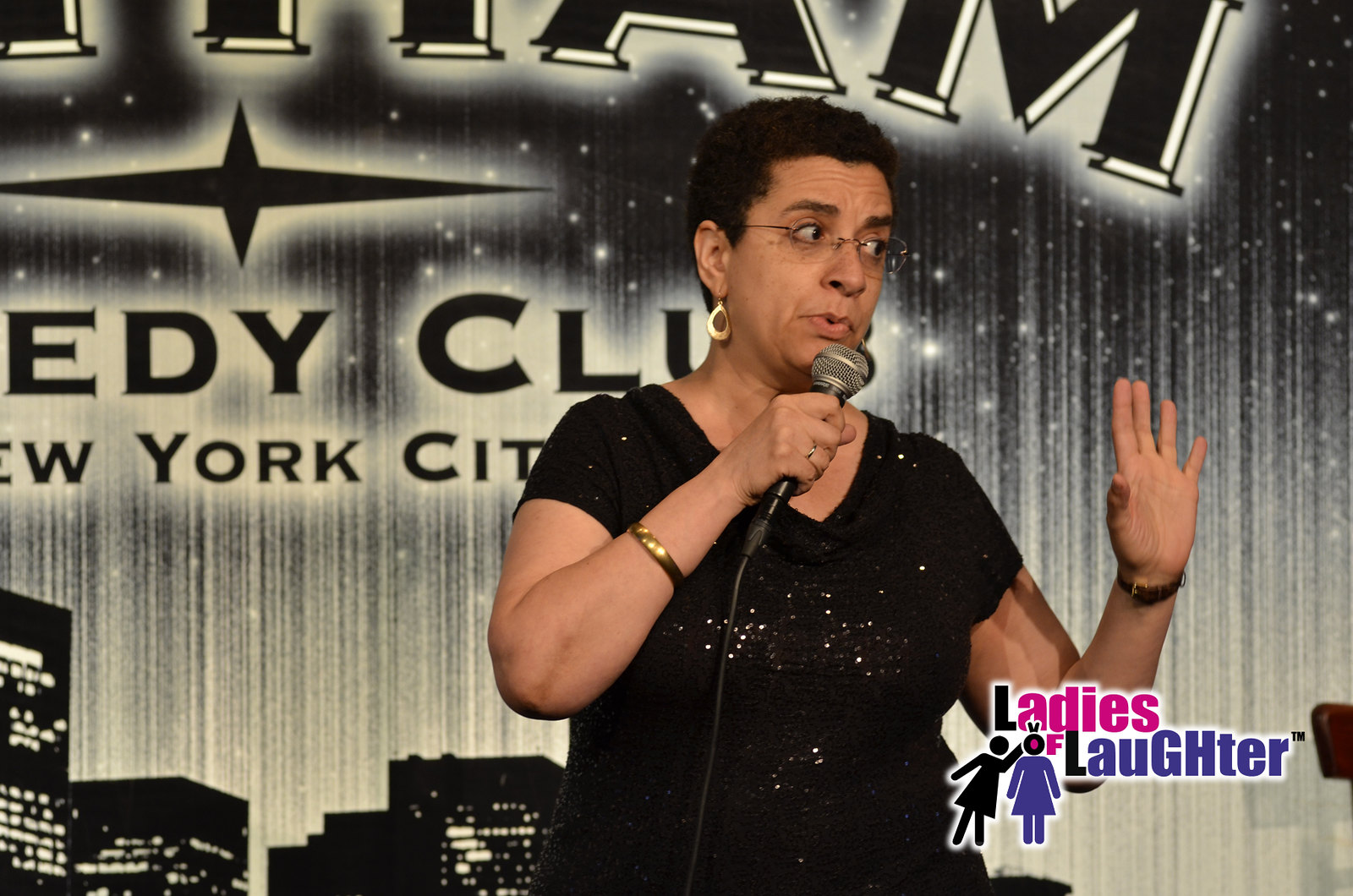In this striking paint-like photograph, a woman in her 40s, identified as an African-American comedian, commands the stage with a poised and confident demeanor. She has short, curly black hair and light brown skin, and she is dressed in a sparkly black V-neck dress. Her ensemble is complemented by gold earrings, a gold bracelet, a wristwatch, and glasses. She is holding a microphone with her right hand and gesturing thoughtfully with her open left hand, as she gazes slightly downward.

The backdrop features a gray curtain with a partially visible city skyline and the words "Comedy Club New York City," though parts of the phrase are cut off. Above these words, there are two diamond shapes forming part of the club's logo. The background also includes black high-rises with white lights, giving it a night-sky ambiance. In the bottom right-hand corner of the image, there is a logo for "Ladies of Laughter," featuring two stick-figure women. The text is colored red and purple, with 'Ladies' in red (except for the 'L') and 'Laughter' in purple.